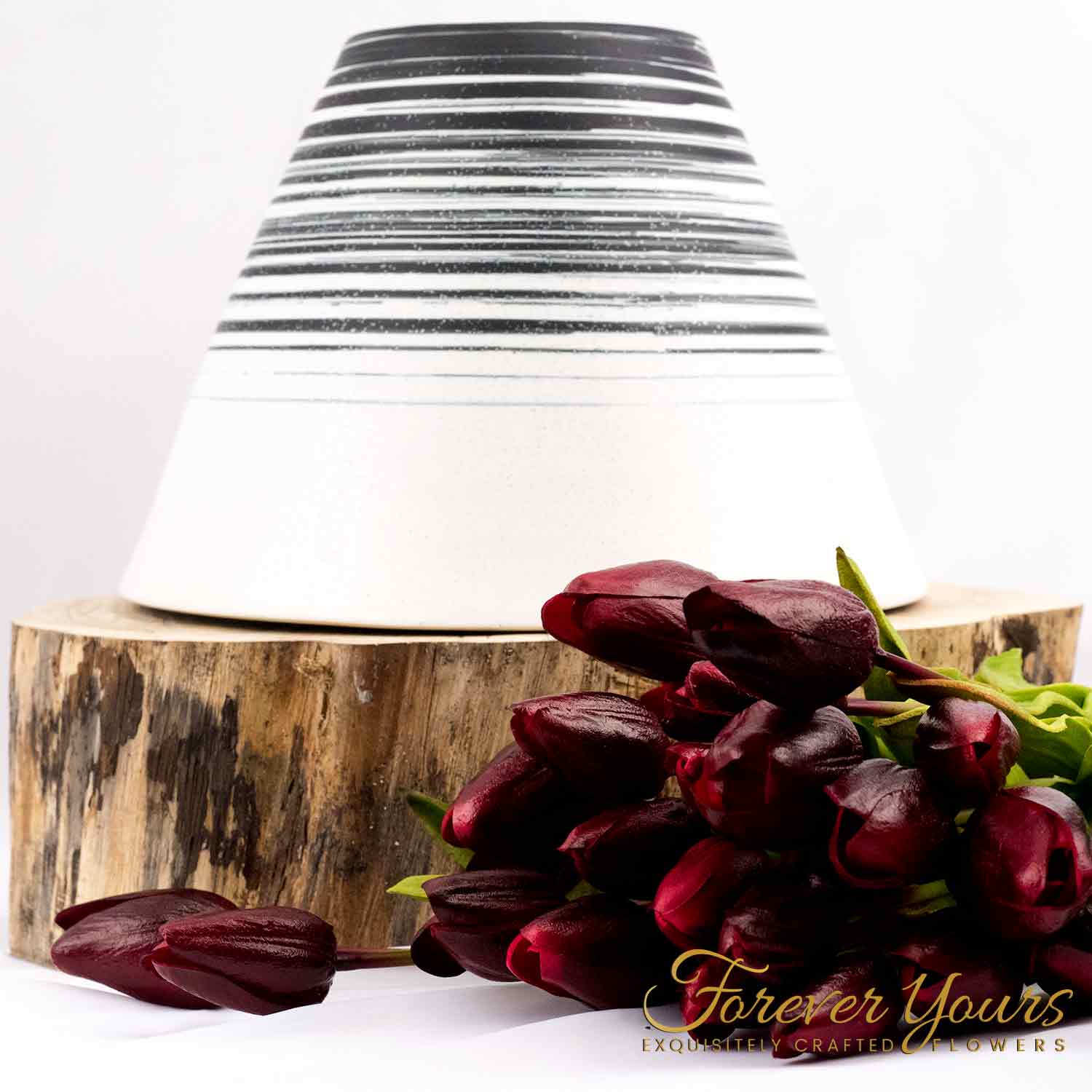In this captivating photograph, there is a bouquet of deep, burgundy red roses, adorned with lush green stems and leaves, situated in the foreground. The roses, yet to bloom, appear as elegantly crafted buds, presenting a rich maroon hue. Two additional rosebuds lie separately in the front, complementing the arrangement. Behind this alluring floral display is a cylindrical block of wood, reminiscent of a tree trunk slice, on top of which sits a distinctive white lampshade. The lampshade features eye-catching black stripes that elegantly descend halfway down. The background is a stark, clean white, adding to the visual emphasis on the arrangement. In the bottom right corner, elegantly written in gold cursive and print, the text reads: "Forever Yours, Exquisitely Crafted Flowers," suggesting a polished advertisement for a premium flower shop.